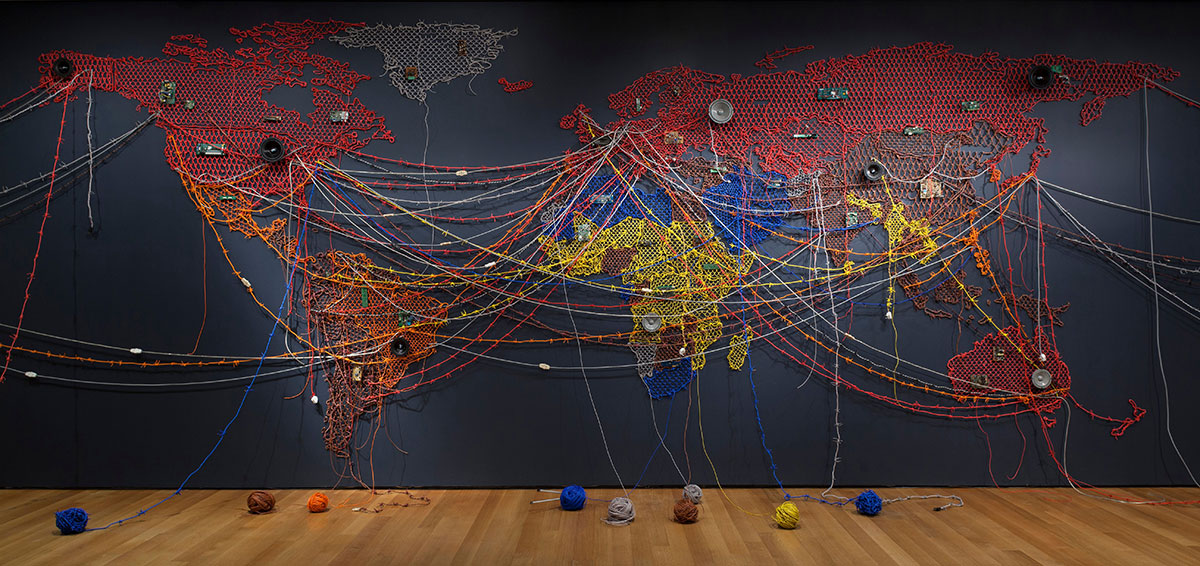This color photograph features a dark blue wall adorned with an intricate and unique world map created entirely from yarn. The continents are meticulously outlined using different colored yarn: North America and Australia are rendered in red, Central America and South America in orange, Africa predominantly in yellow with hints of blue, and Asia primarily in red. The map omits Antarctica. Numerous strings stretch between the continents in arched and looped patterns, creating a web-like effect that connects various parts of the world. The yarn is attached to the wall and unravels down to the wooden floor, where several balls of yarn are scattered, completing the elaborate art installation. There are no visible words, writing, people, or animals in the image.